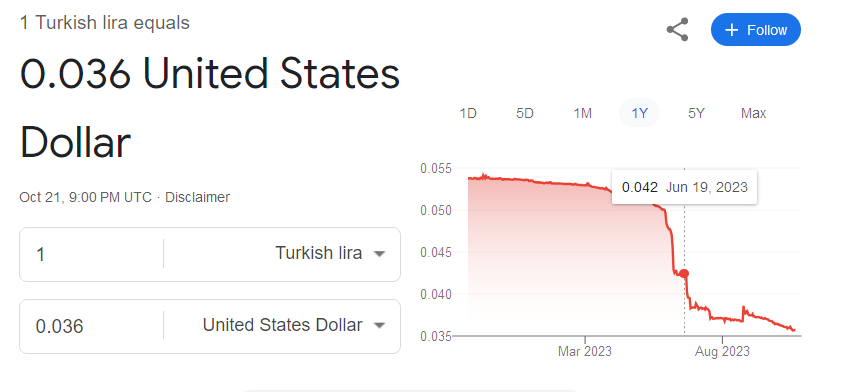This image is a screenshot of a Google search result for the exchange rate between the Turkish Lira (TRY) and the United States Dollar (USD). At the top, it displays "1 Turkish Lira equals 0.036 United States Dollars." The text for Turkish Lira is in gray, while the USD is prominently displayed in dark black and blue. On the right side of the screenshot, there is an option to share the result, as well as a "Follow" button.

The timestamp for this data is October 21st at 9 p.m. UTC. A disclaimer is also present, indicating the rates are subject to change. Below the initial exchange rate information, it reiterates, "1 Turkish Lira equals 0.036 United States Dollars."

To the right of this information is a graph showing the historical worth of the Turkish Lira against the USD. The graph provides selectable time scales: 1 day, 5 days, 1 month, 1 year, 5 years, and max. The 1-year time scale is selected, highlighted by a gray box, and the line graph inside is blue.

Examining the graph, the highest value shown is 0.055 USD, while the lowest is 0.035 USD. Specific timestamps like March 2023 and August 2023 are marked, with June 19th, 2023 highlighted, showing an exchange rate of 0.042 USD. The graph begins around 0.052 USD and depicts a significant decline around May to June 2023, where it drops to 0.035 USD and remains in that range for the remainder of the displayed timeline.